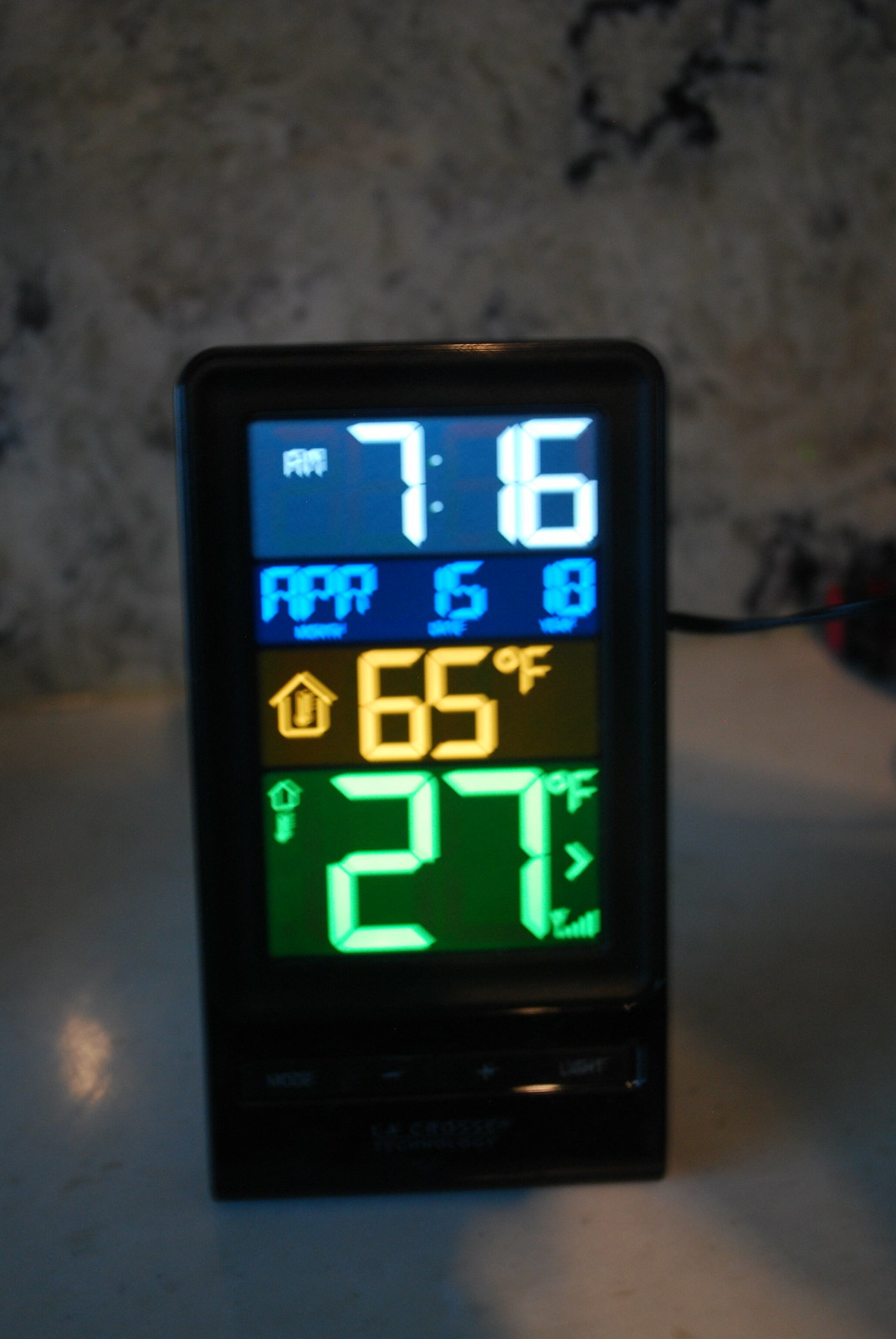The image depicts a digital weather station displayed in a sleek black case, standing upright on a white kitchen countertop against a splash wall. The top section of the display shows the time "7:16 AM" in white letters with a blue backdrop. Below it, the date "April 15th, 2018" is displayed in blue letters. The next section features a house icon beside the temperature "65°F," presumably indicating the indoor temperature. The bottom section reads "27°F" with an arrow, likely denoting the outdoor temperature. The device casts a shadow on the countertop, with light glaring off its surface, suggesting a light source is on in the background.